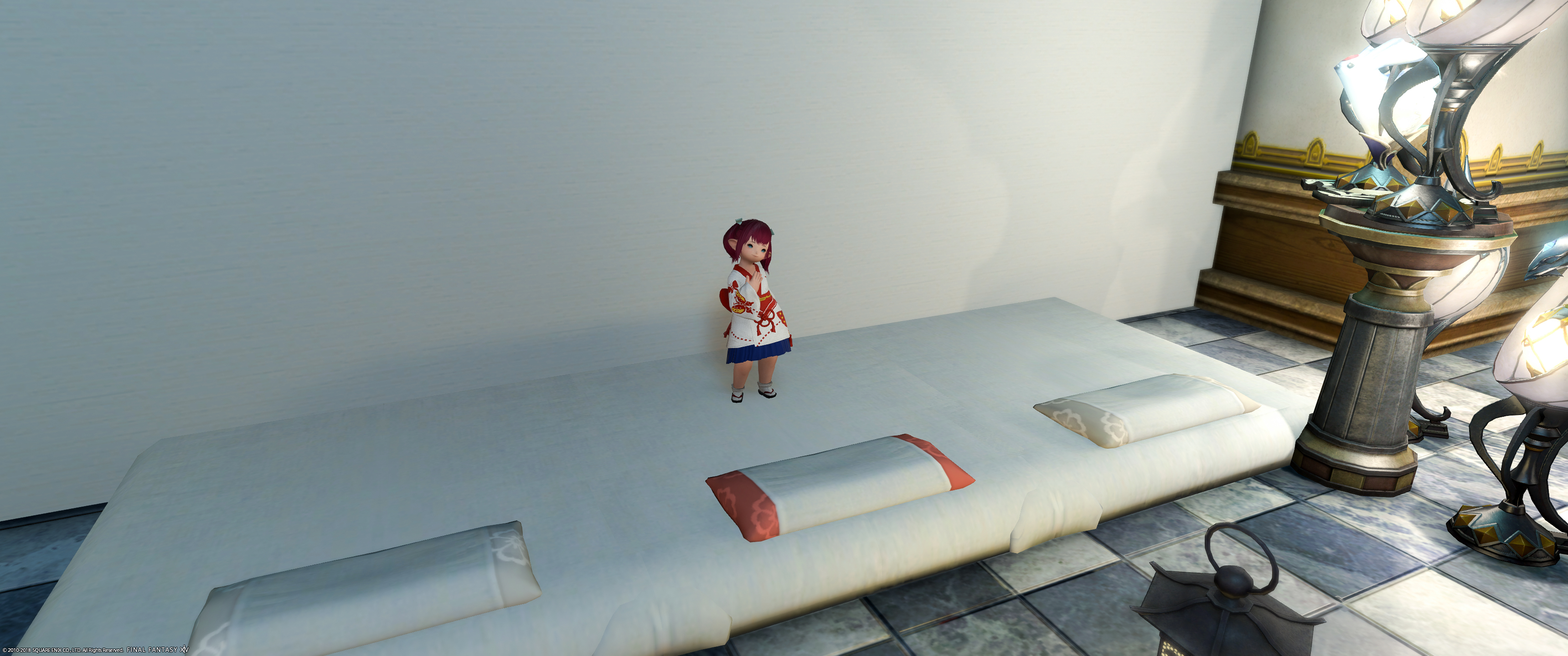This is a color photograph featuring a detailed setup centered around a white rectangular mattress placed on a floor of dark blue and blue square tiles. At the center of the mattress stands an Asian figurine resembling an elf, adorned in traditional attire—a white kimono-style top with a red graphic design and a plain blue skirt—giving it a bell-like appearance. This doll, noted for its disproportionate short legs compared to its adult or adolescent representation, has brown-red hair. 

In the foreground on the left, there is the top of an intricate Asian lantern. To the right of the mattress, floor lights cast a soft glow, illuminating the scene subtly from below. On the mattress, near its edge closest to the viewer, lie three very flat rectangular pillows, seemingly placed for kneeling, further enhancing the ritualistic setup around the figurine. There is no text or additional markings on the photograph, leaving the viewer to contemplate the serene yet puzzling tableau.